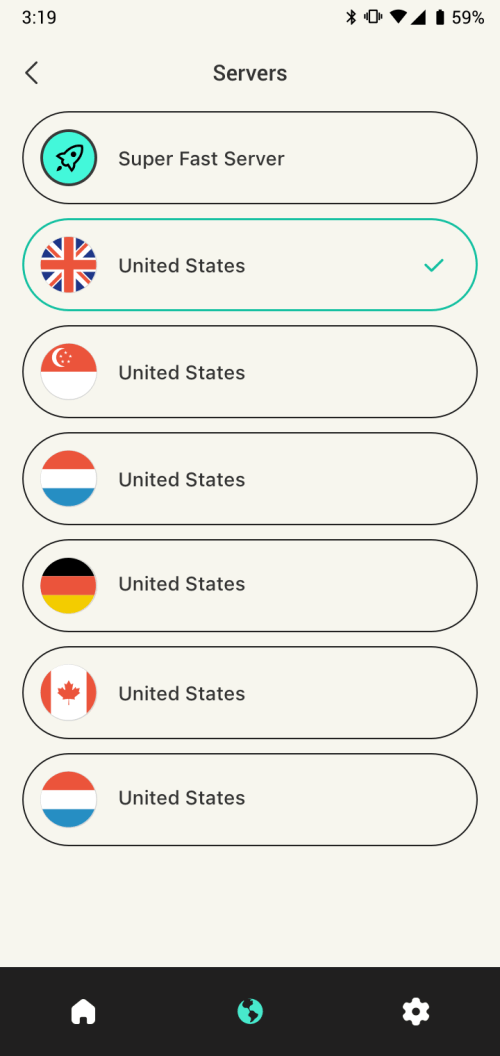In the top-left corner of the screen, the status bar displays several indicators: 'C318' is shown, along with icons for Bluetooth, a vibrating alert, a strong Wi-Fi connection, full cell signal, and a battery level at 59%. Next to a left-pointing arrow, the text reads "BlackTek servers". Below that is an oval shape containing the text "Super Fast Server", and to its left, there is a blue-colored rocket ship icon.

Further below, there is information about various server locations. The first entry lists "United States" with an accompanying British flag and a green check mark, indicating it is selected or active. The next oval states "United States" again but displays a Singaporean flag next to it, implying a discrepancy or error. The following entries list countries with the United States repeatedly mentioned alongside incorrect or mixed flags such as Germany (black, red, yellow) and Canada (red, white) in a red oval. Additionally, another "United States" entry is displayed with a red, white, and blue theme.

At the bottom of the screen, there is a black section that appears to contain an image or graphic of a building, a planet, and a gear, suggesting some sort of control or configuration options.